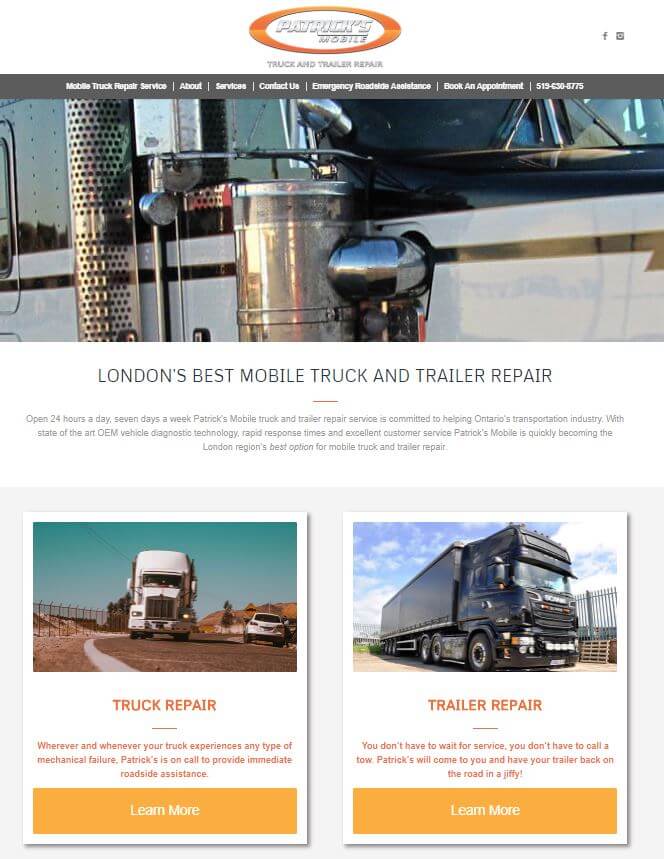This detailed caption provides a thorough description of the promotional imagery for "Patricks Mobile Truck and Trailer Repair" service.

---

Screenshot Description: 

**Header:**
A sleek gray bar stretches across the top of the image, displaying in white text: "Mobile Truck Repair Service | Services | Contact Us | Emergency Roadside Assistance | Booking Appointment | 519-630-8775". On the top right, small Facebook and Instagram icons signal social media presence.

**Main Logo:**
The logo text "Patricks" features a stylish metallic appearance with a gradient from gray at the top to white in the center, giving it a hollow effect. An elegant line extends from the "R" underlining "X", with "Mobile" placed beneath this line. Below the logo, a dark-to-light orange gradient oval houses the text "Truck and Trailer Repair".

**Promotional Banner:**
A large, high-resolution close-up image of a semi-truck cab dominates the center. This cab, viewed from the passenger side, is white on the bottom and black on the top. Notable elements include the smokestack and another unidentified silver cylinder. A bold black line resembling a lightning bolt adds dynamic flair to the front of the cab.

**Tagline and Service Information:**
Underneath the image, set against a white background, is the compelling tagline in capital letters: "London's Best Mobile Truck and Trailer Repair". A short gray horizontal line follows, leading to the service details: "Open 24 hours a day, 7 days a week. Patricks Mobile Truck and Trailer Repair Service is committed to helping Ontario's transportation industry. With state-of-the-art OEM vehicle diagnostic technology, rapid response times, and excellent customer service, Patricks Mobile is quickly becoming the London region's best option for mobile truck and trailer repair."

**Service Highlights:**
Against a light gray background, two promotional cards further emphasize the service offerings:

1. **Truck Repair:**
   The left card features an image of a white semi-truck approaching the viewer, with a white station wagon beside it and a person standing outside the passenger door. The scene includes a tall fence, trees on a hill, and a dirt road under a blue sky. In bold orange capital letters, it reads "TRUCK REPAIR". Below, a short horizontal line precedes the text: "Wherever and whenever your truck experiences any type of mechanical failure, Patricks is on call to provide immediate roadside assistance." An orange "Learn More" button invites further exploration.

2. **Trailer Repair:**
   The right card showcases an image of a black semi-truck with a trailer, positioned against a backdrop of green grass, a bridge, and a tall fence. Featured prominently is a wooden pallet. In bold orange capital letters, it states "TRAILER REPAIR". Below a horizontal line, it continues: "You don't have to wait for service, you don't have to call a tow. Patricks will come to you and have your trailer back on the road in a jiffy!" An orange "Learn More" button is positioned below.

This richly detailed emblazonment captures not only Patricks Mobile's offerings but their dedication to supporting Ontario's transportation industry with swift, efficient, and professional service.